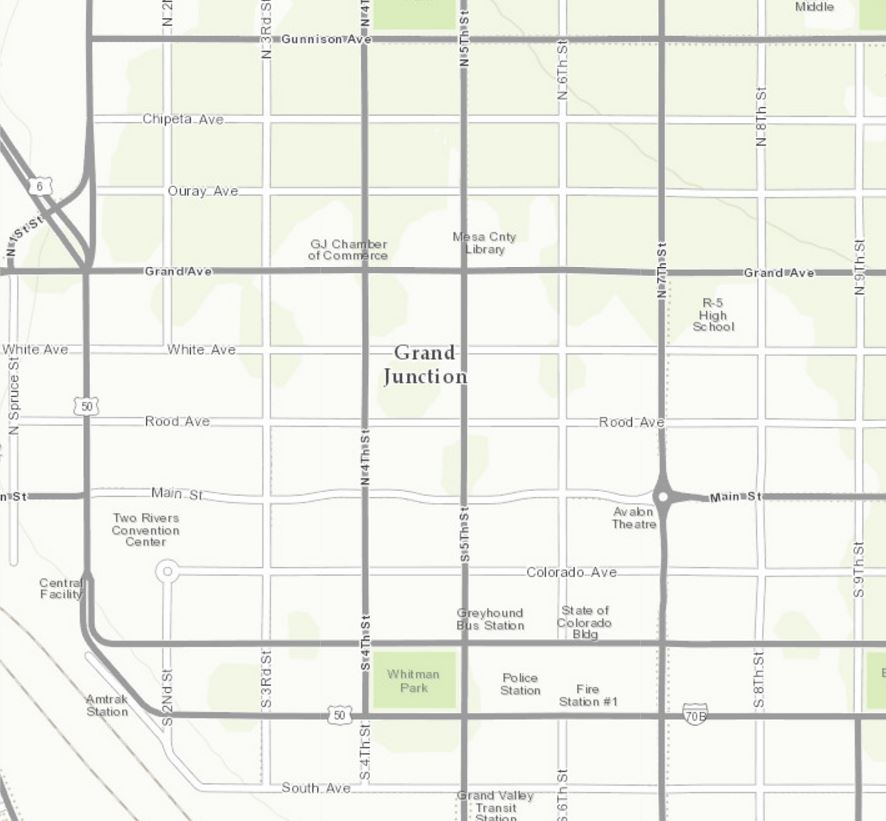The image depicts a detailed street map of Grand Junction, characterized by a predominantly grid-like layout with minimal curved streets. Major thoroughfares are indicated by a darker gray tone, distinguishing them from the lighter-toned surface streets. The labeled streets from top to bottom include Gunnison Avenue, Chapita Avenue, Oray Avenue, Grand Avenue, White Avenue, Rood Avenue, Main Street, Colorado Avenue, with two unlabeled streets following, and South Avenue at the bottom. From right to left, the streets are labeled as South 2nd Street, South 3rd Street, South 4th Street, South 5th Street, South 6th Street, North 7th Street, North 8th Street, and North and South 9th Street. Additionally, the outer edges of the map feature North 1st Street, North Spruce Street, and an Amtrak station is located in the bottom left corner.